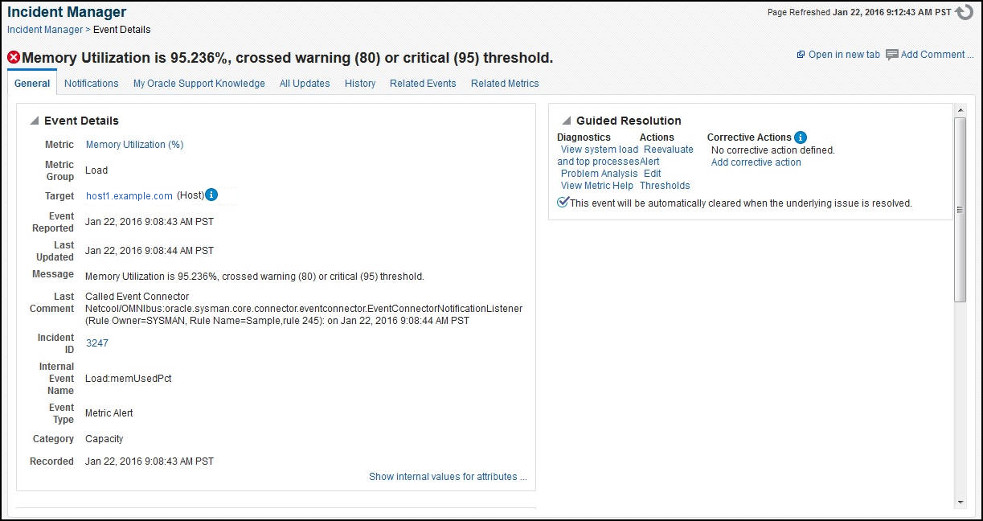[Incident Management Interface Screenshot, January 22, 2016]

This image displays a detailed screenshot of an incident management interface. At the top of the interface, several tabs are visible: "General," "Notifications," "My Oracle Support Knowledge," "All Updates," "History," "Related Events," and "Related Metrics." Below these tabs, the screen shows critical information about an event, particularly focusing on memory utilization data.

The memory utilization at the time of the screenshot is recorded at 95.236%, which has surpassed the warning threshold of 80% and reached the critical threshold of 95%. This significant level of memory usage is flagged as a metric alert within the system.

The section labeled "Event Details" provides further specifics, indicating the date of the incident as January 22, 2016. The event has been assigned to an Event Coordinator and involves several entities, including Net Call, Omnibus, the bus system, Oracle, and a System Manager. The type of event is classified as a Metric Alert, pointing to a potential capacity issue within the system.

An additional note on the interface explains that the event will automatically be cleared once the underlying issue has been resolved, indicating a proactive monitoring and resolution system.

The importance of image clarity is highlighted, suggesting that the original screenshot may not be very clear and requires magnification, hinting that improvements in image quality would aid in better analysis and understanding of such critical information.